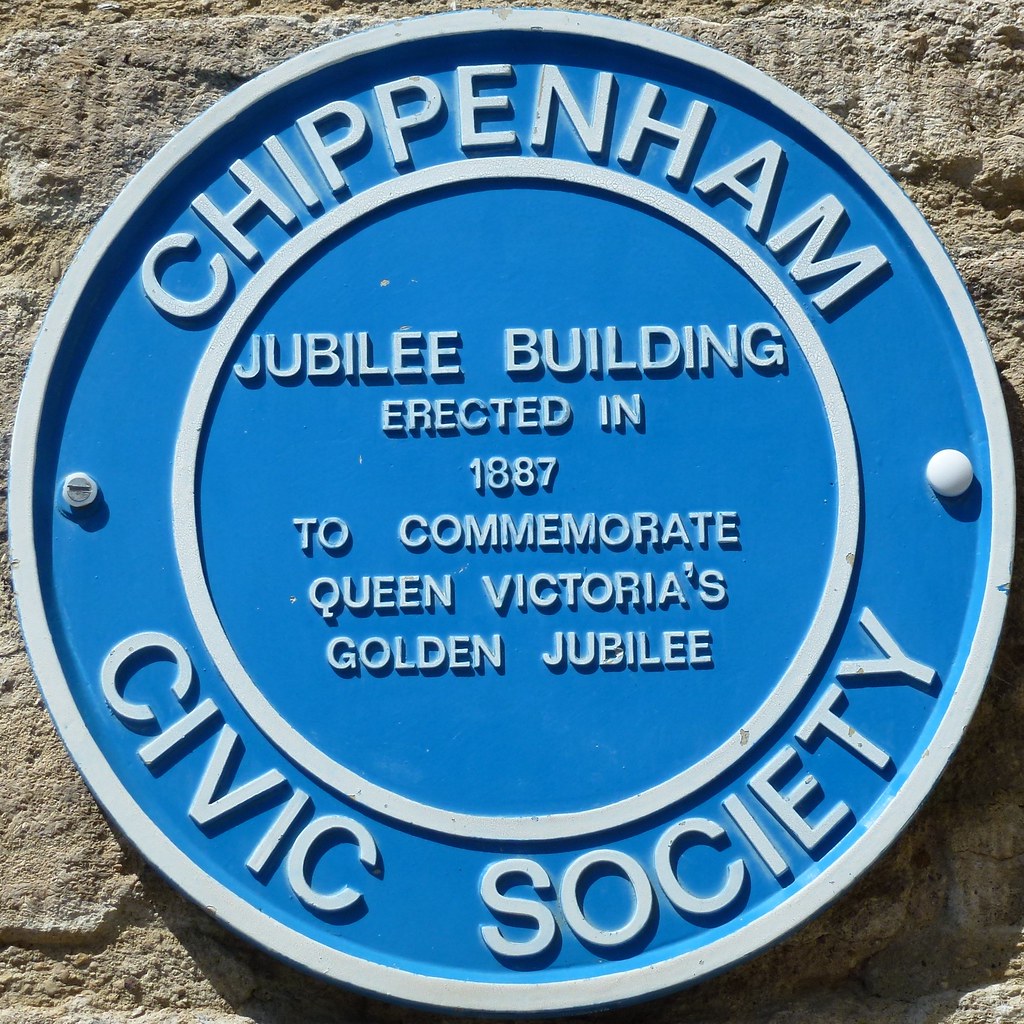The image captures a professionally-taken, outdoor scene of a metallic marker against a brownish-gray stone wall. The focal point is a blue, circular metal sign. This sign features two concentric circles outlined in white. In the outer circle, the text "CHIPPENHAM CIVIC SOCIETY" is displayed in white. Within the inner circle, the text reads: "Jubilee Building erected in 1887 to commemorate Queen Victoria's Golden Jubilee," also in white. The marker is affixed to the wall with a white-headed nail on the right side and a simple silver tack on the left. Bathed in sunlight, the image sharply captures the vivid blue, white, and stone hues, conveying a sense of stillness and precision, devoid of people, plants, or animals.